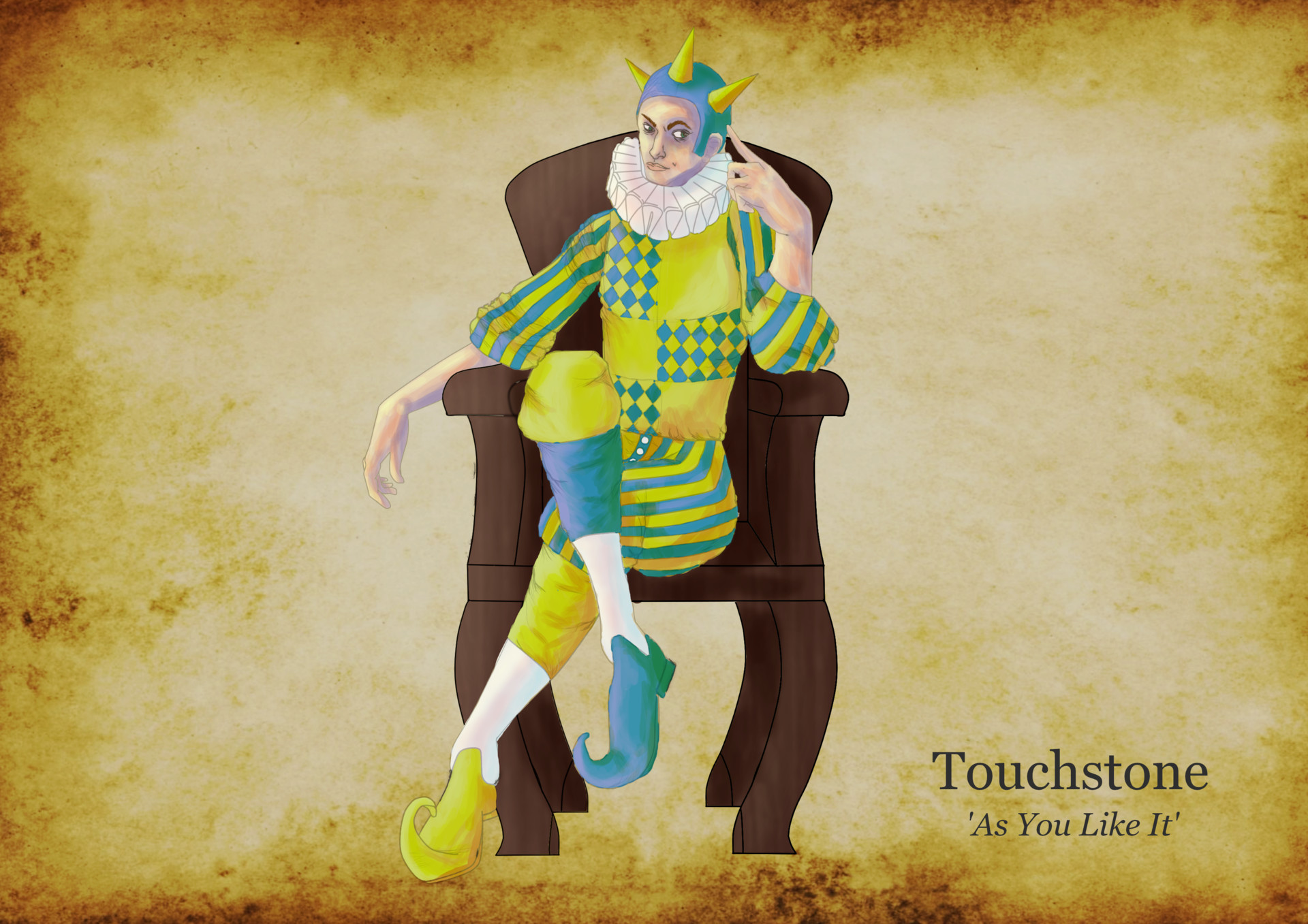This drawing, presented on weathered and rust-stained paper, exudes a sense of aged elegance. In the lower right corner, the black font script identifies the subject as "Touchstone," with the subtitle "As You Like It" beneath it. At the heart of this artwork is a jester, regally seated on a brown throne. His expression is stern, with an almost angry demeanor. The jester is adorned in an elaborate blue hat, distinguished by its three spikes tipped with yellow. His right hand is placed thoughtfully, with his pointer finger resting on the side of his forehead. He wears a quintessential puffy white collar, adding to his distinguished yet playful appearance. The jester's jumpsuit is a whimsical patchwork of yellow and blue stripes, diamond patterns, and checkered sections. His attire is asymmetrical, featuring a blue cuff on one pant leg and a yellow cuff on the other, complemented by white stockings. His shoes, each curling up at the toes, are mismatched in color—one blue and one yellow—completing his eccentric ensemble.